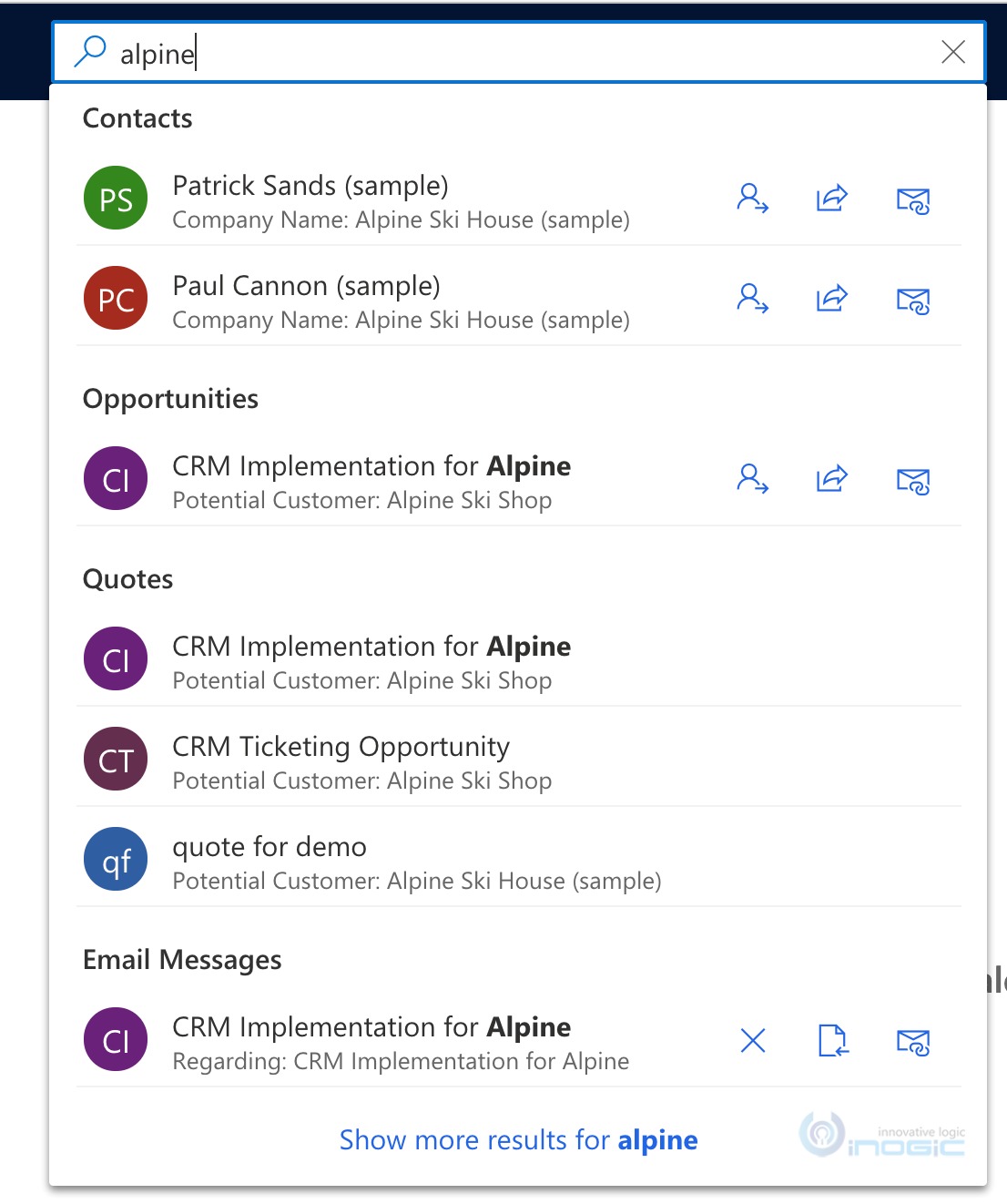This image portrays a clean, predominantly white interface, featuring a search being conducted on what appears to be a contacts or CRM page. At the top of the image, there is a subtle navy blue border. Central to the interface is a prominent white search bar, accentuated with a light blue border and a blue magnifying glass icon within it. The search term displayed is "Alpine."

Below the search bar, the results are listed methodically:

1. Contacts:
   - Patrick Sands, associated with "Sample Company Name" and "Alpine Ski House (Sample)."
   - Paul Cannon, associated with "Sample Company Name" and "Alpine Ski House (Sample)."

2. Opportunities:
   - CRM Implementation for Alpine, categorized as a potential customer, "Alpine Ski Shop."

3. Quotes:
   - CRM implementation for Alpine, listed as a potential customer, "Alpine Ski Shop."
   - CRM ticketing opportunity, categorized as a potential customer, "Alpine Ski Shop."
   - Quote for a demo, listed for potential customer, "Alpine Ski House (Sample)."

4. Email Messages:
   - Various CRM implementation communications relating to "Alpine."

At the bottom of the search results, there is an option to "Show more results for Alpine."

Lastly, a watermark is visible, displaying the text "INOGIC" in a lighter blue color, with lowercase 'i's and the rest of the letters in uppercase.